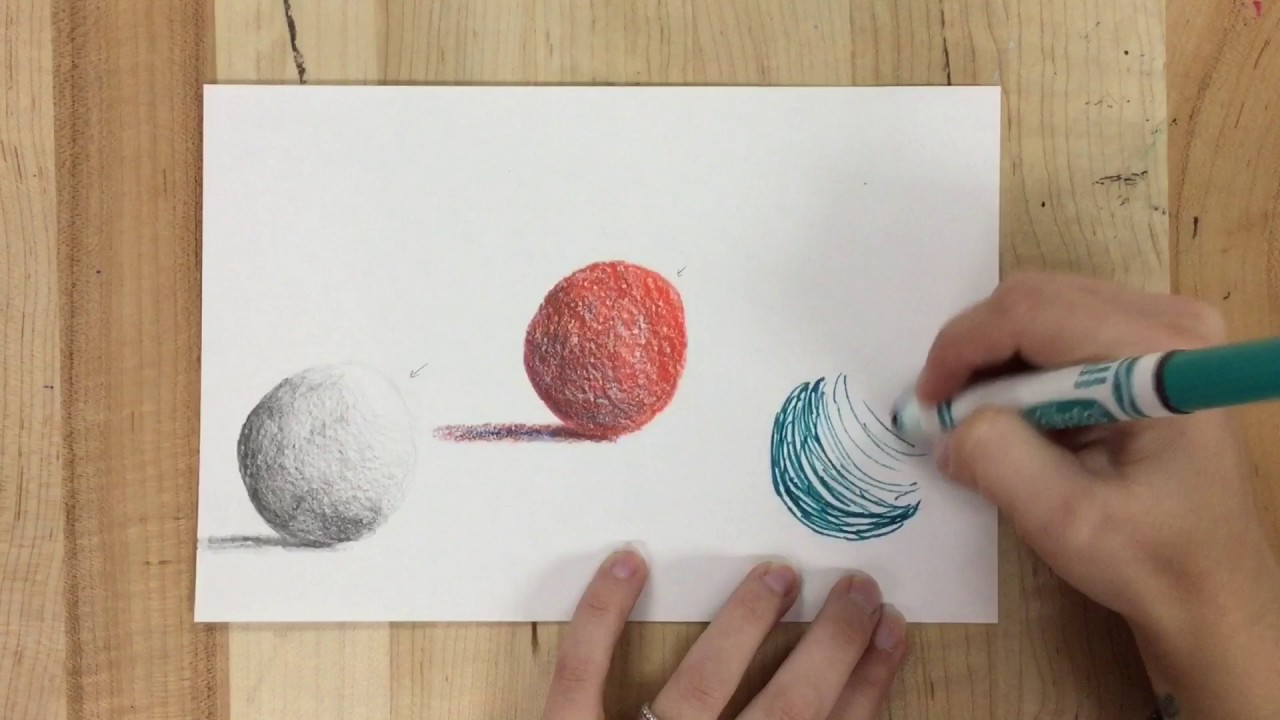The rectangular image, approximately twice as wide as it is tall, features a light-colored wooden table as the background, marked with a visible crack running from the top left toward the bottom middle. In the foreground, two hands emerge from the bottom edge of the frame. One hand, on the bottom right, is clasping a turquoise Crayola marker, while the other hand, positioned in the center, reveals a barely visible ring on the ring finger.

The hands are drawing on a sheet of white computer paper oriented horizontally. On the left side of the paper, a ball-shaped image shaded in gray appears. In the center of the paper, another ball has been fully colored in red with visible texture, casting a shadow on its left side. The artist is in the process of sketching a partially completed circular design on the right side of the paper using the turquoise marker, showing a sequence of half-circle lines that suggest the form of another ball. The shaded and colored elements extend from the bottom left towards the top right of the image, showcasing the artist's progression from left to right.